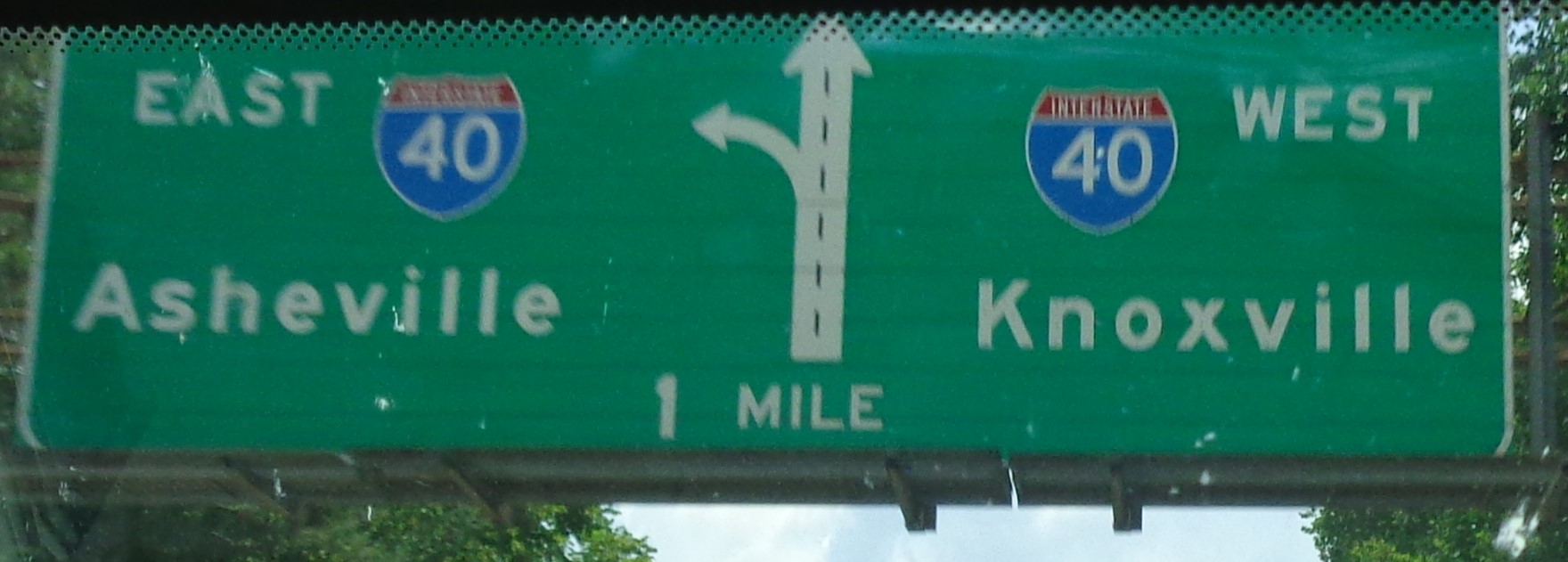This is a close-up photograph of a large green directional highway sign, the kind typically suspended over a freeway to guide drivers when there is an approaching lane split or exit. The sign is supported by a black metal post and is edged in white with white lettering. At the top of the sign, there are traditional red, white, and blue interstate shield logos for Interstate 40. The red bar at the top of these shields reads "Interstate," and the blue field below it displays the number "40" in white.

In the center of the sign, there's a diagram indicating a road with a large white arrow pointing straight and another arrow veering to the left, accompanied by a notation that the split is coming up in one mile.To the left of the sign, it instructs that East Interstate 40 leads to Asheville, while to the right, it indicates that continuing straight on Interstate 40 West heads towards Knoxville. The background of the image features a bit of sky visible at the bottom, completing the context of this directional sign on a divided highway.